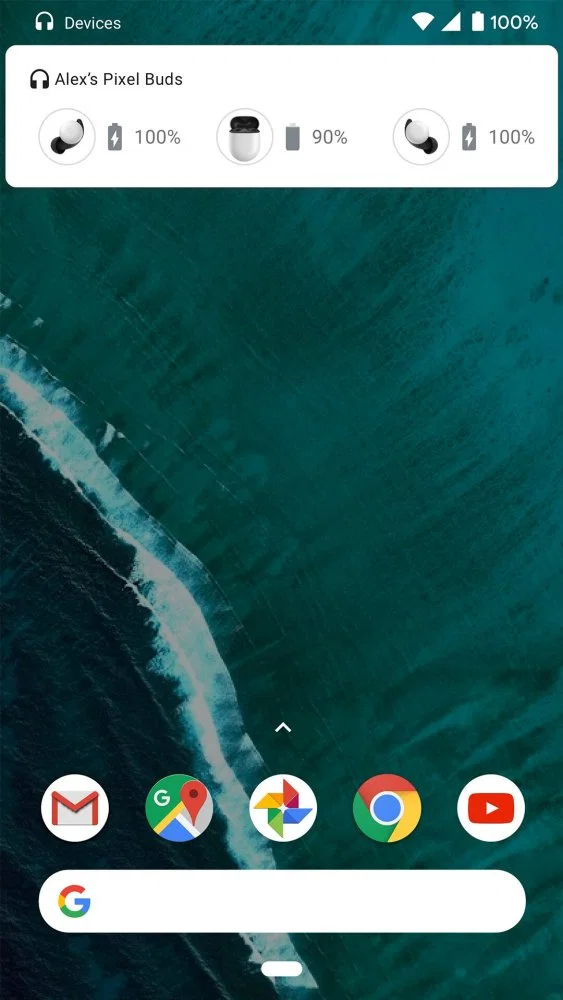The image depicts a smartphone interface with several key elements and indicators. At the top left corner, there is a "Devices" label accompanied by a small white icon of headphones. In the top right corner, standard status icons are shown, including a Wi-Fi symbol, reception bars, a battery icon displaying full charge, and the percentage "100%" written in white.

Below the status icons, there is a white rounded rectangle containing the text "Alex's Pixel Buds" in black. Within this rectangle is a small black icon of headphones. Beneath this section, the interface displays the Pixel Buds themselves, illustrated with black and white coloring inside a circular frame, accompanied by a battery icon showing a full charge with a lightning bolt symbol, and the text "100%".

Next, the case of the Pixel Buds is shown, depicted as having a black interior and a white exterior, along with a battery icon showing "90%". Another indicator represents the second earbud, also displaying a battery icon with a lightning bolt symbol and "100%". 

The phone's background features a wave-like design with shades of blue and green. At the bottom of the screen, there are multiple app icons, including Gmail, Maps, Photos, Google Chrome, and YouTube. Below these icons, a white search bar is clearly visible.